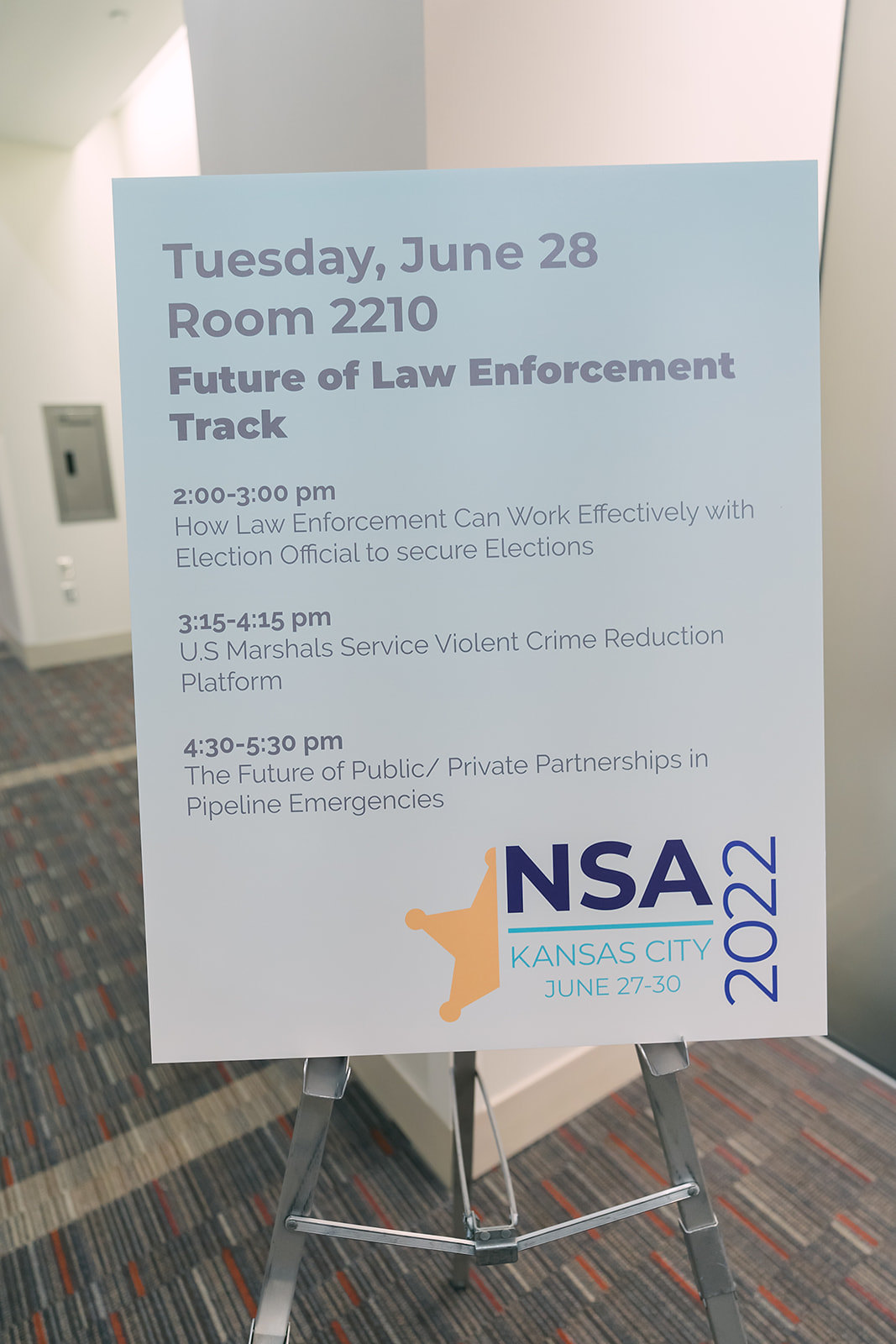The image depicts a rectangular, slightly faded photograph taken indoors, likely in a conference area or hotel hallway. The walls are white, and the flooring is thin, gray carpet with red and white stripes. Centered in the hallway is a silver easel stand holding a large white poster board. The poster features a schedule for "Tuesday, June 28th, Room 2210, Future of Law Enforcement Track," with three events listed in light gray text. From 2:00 to 3:00 p.m. is "How Law Enforcement Can Work Effectively with Election Officials to Secure Elections." From 3:15 to 4:15 p.m. is the "U.S. Marshals Service Violent Crime Reduction Platform." From 4:30 to 5:30 p.m. is "The Future of Public-Private Partnerships in Pipeline Emergencies." At the bottom right of the poster, there is a logo with a yellow, half-star sheriff’s badge next to "NSA" in bold blue text. Below this, a light blue line underlines "Kansas City, June 27th-30th," with "2022" written vertically in blue on the right side. A metallic fire extinguisher is also visible, adding to the institutional feel of the hallway.